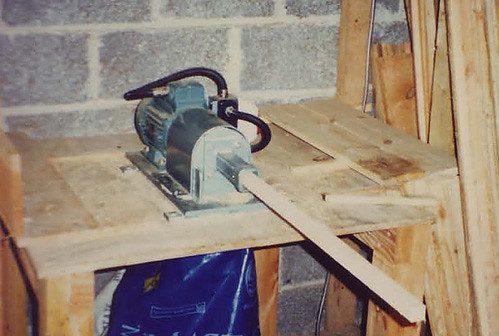This vintage photograph, likely from the 70s or 80s, showcases a substantial power tool used in woodworking, possibly a sandblaster or similar device meant for smoothing wood. The apparatus, predominantly bluish-gray with a black hose or pipe extending from it, is mounted on a sturdy wooden table. Scattered on the table and propped against a gray cinder block wall are several slabs of wood, including 2x4s. Tucked beneath the table is a noticeable blue plastic bag or object, adding to the scene's rustic workshop ambiance. The intricate setup of wires and components, along with the wood piece inserted into the tool, evokes a sense of the manual craftsmanship involved in its operation.